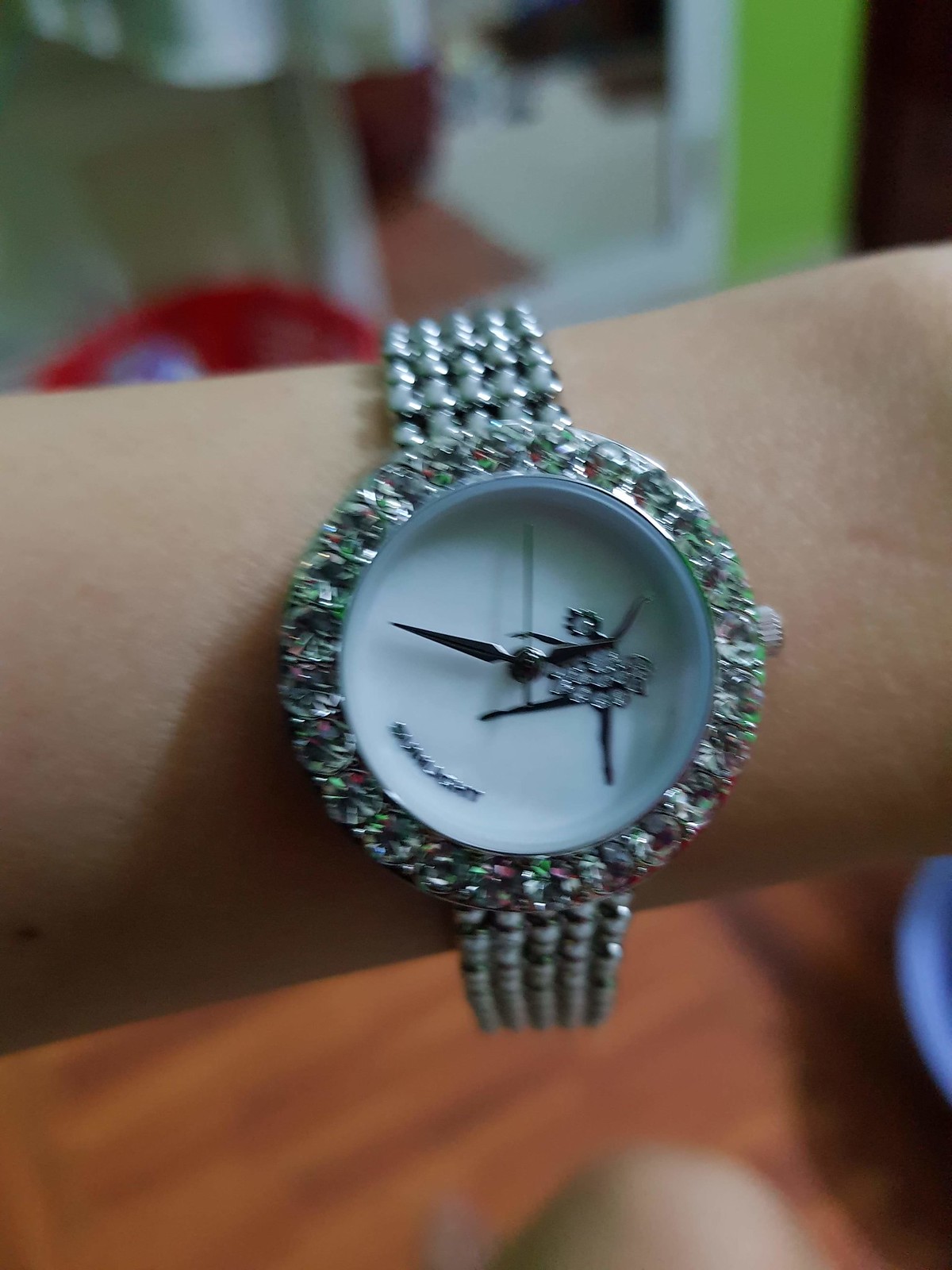This is a portrait-style, close-up image of a woman's wrist adorned with an ornate and elaborate wristwatch. The person's skin is white, and the image captures from the middle of her forearm to just past her wrist, but does not include her hand. The watch itself is very fancy, featuring a strap made of silver ball beads encrusted with various colored gems, including pink, yellow, white, and green. The face of the watch is solid white with two black hands indicating the time, around 2:45. 

At the center of the watch face, a detailed ballerina figure, adorned with a gem-studded tutu, poses gracefully with one leg on the floor and the other outstretched. Although there's some text on the watch face, it is too blurry to read. The image quality is low and out of focus, contributing to a slightly unclear view of the intricate details.

The background of this photograph is blurred, but hints at an indoor setting. Visible elements include what might be a red clothes basket and various colors like light green, blue, maroon, dark peach, tan, cream, and a knee protruding at the bottom of the image. The floor beneath the wrist appears to be a dark brown or golden-brown color. Overall, the composition emphasizes the dazzling, gem-encrusted watch against a kaleidoscope of blurred background colors.